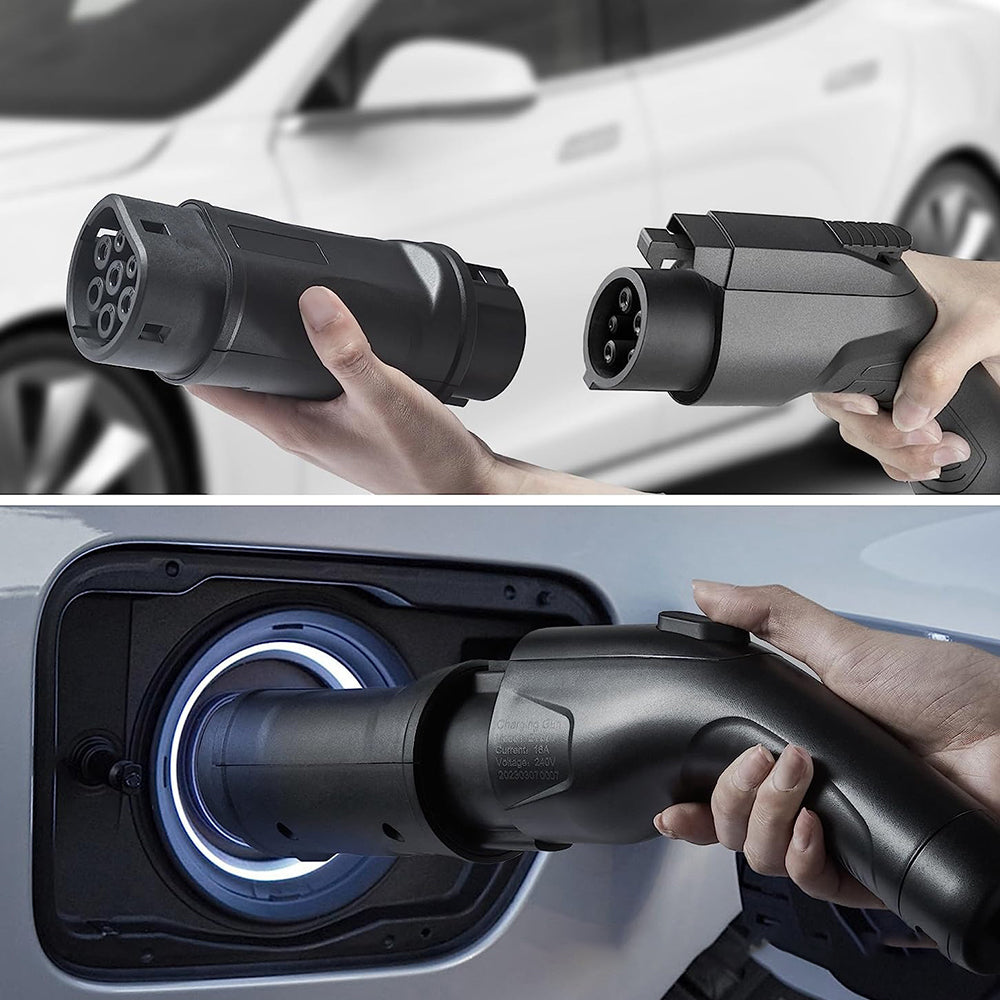The image is a two-part advertisement demonstrating the process of charging an electric vehicle. In the top photograph, a person is seen using both hands to connect two components of an electric car charger. The right hand holds the main nozzle, while the left hand aligns an attachment to plug into it. The electric charger, predominantly black with seven circular connections, stands out against the backdrop of a white sedan. In the lower photograph, the now-assembled charger is plugged into the car’s charging port, reminiscent of a fuel tank slot in conventional vehicles. The charging port emits a blue-white light, indicating active charging, with visible details such as the voltage rating of 240 volts and current of 18A. The charger’s components and the surrounding port light provide a stark contrast of black, white, and blue hues, underlining the modernity and functionality of the electric charging setup.